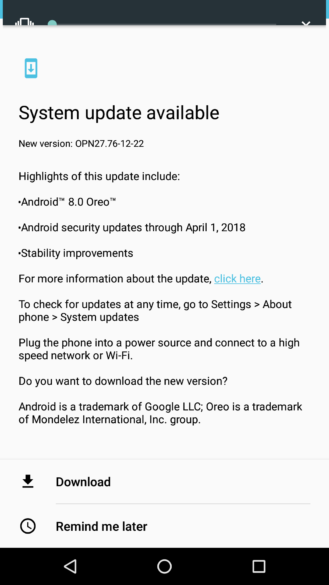This screenshot features a clean, solid white background with a prominent black banner at the top, serving as a header. Below this header, a blue rectangle with a downward-pointing arrow draws attention to the main message. The essential information is encapsulated in bold black text that reads, "System Update Available: New Version OPN27.76-12-22." 

Key highlights of this update are meticulously detailed, including:
- Upgrade to Android 8.0 Oreo
- Android security updates up until April 1, 2018
- Various stability improvements

Additionally, a clause prompts users to click a link for more information about the update. It also provides instructions on how to manually check for updates at any time by navigating to Settings, then About Phone, followed by System Updates. The screenshot concludes with a crucial reminder to plug the phone into a power source and connect to a high-speed network or Wi-Fi to ensure a smooth update process.